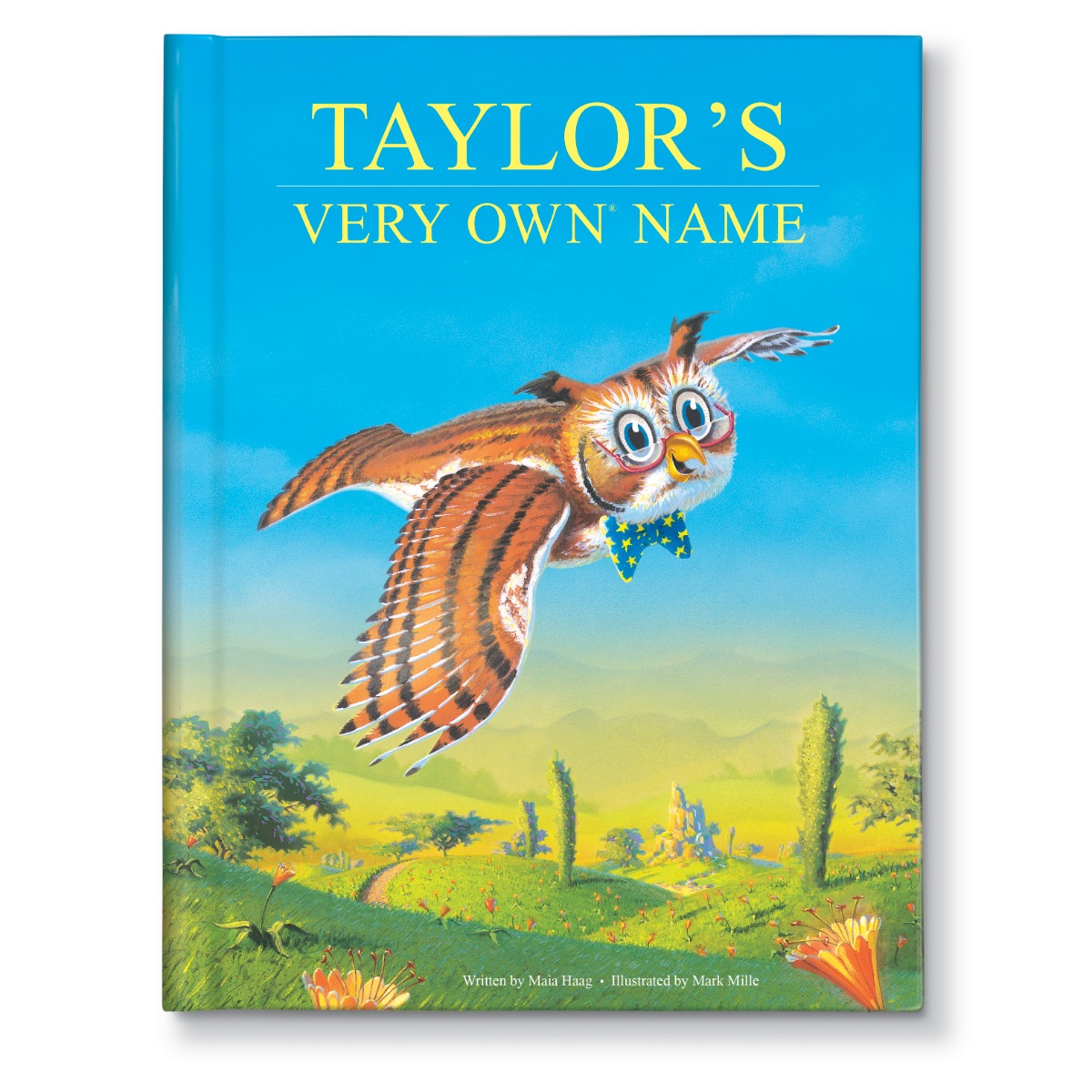The cover of the children's book "Taylor's Very Own Name," authored by Maya Haag and illustrated by Mark Mille, is vibrant and captivating. At the top in bright yellow all-capital letters, the title "Taylor's Very Own Name" stands out against a clear blue sky. The main image features a whimsical owl in mid-flight above rolling green hills dotted with plants and flowers. The owl is distinctively black and orange-striped, wearing a blue bowtie adorned with yellow stars and half-moon glasses with pink rims. Its blue eyes and white eyelashes are prominently displayed, and its ear flaps are orange tipped with black. A dirt pathway meanders through the grassy landscape, leading towards distant mountains that fade into the background. The bright and cheerful depiction of the owl draws viewers' eyes, with its beak giving an impression of a smiling expression. At the bottom of the cover, in small serif font, it reads, "written by Maya Haag" and "illustrated by Mark Mille."